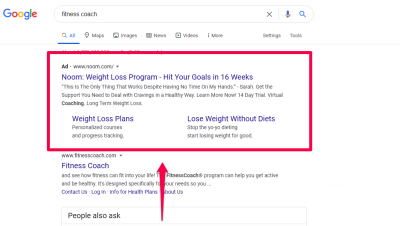The image depicts a Google search results page. The iconic "Google" logo is displayed at the top left in its characteristic multi-color scheme: the first "G" is blue, the "o" is red, the second "o" is yellow, the second "g" is blue, the "l" is green, and the final letter “e” is red. 

In the search bar, the term "fitness coach" has been entered. Adjacent to the right of the search bar, there are three icons: a blue "X" to clear the search, a multicolored microphone icon, and a blue magnifying glass indicating the search action. Below the search bar, various navigation tabs are present: All, Maps, Images, Videos, News, and More, as well as a Settings and Tools option. The "All" tab is currently highlighted in blue.

The first search result is highlighted with a pink rectangle. There is an arrow pointing from the bottom side upward toward a circle, which in turn points to the pink rectangle around the first result. The text within this highlighted result reads: "No weight loss program, hit your goals in 16 weeks. This is the only thing that works despite having no, more than on my hands." However, some text within the highlighted area is cut off and not fully visible. 

Beneath the main result, there are subtopics like "Weight loss plans" and "Lost weight without diet," written in blue, while the descriptions are in black. Another website listed below is "www.fitnesscoach.com," with a subheading simply labeled "Fitness Coach," both written in blue.